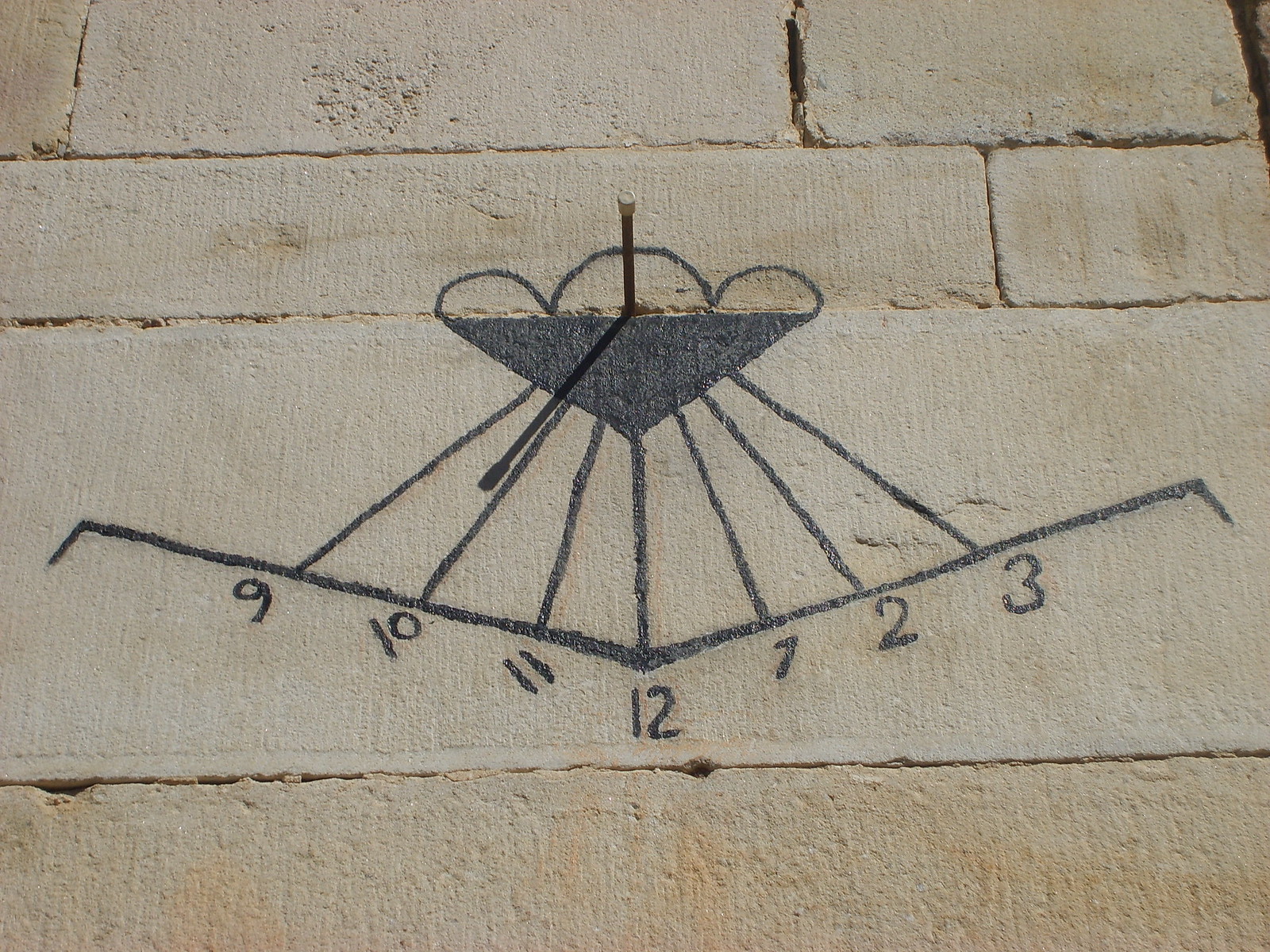This photograph depicts a sundial etched or drawn onto a pale, cream-colored brick surface, likely a brick floor. The bricks vary in size but maintain a rectangular shape, forming a smooth, even surface with visible cracks between them. Central to the design is a fully blackened-in downward-pointing triangle. At the top of the triangle is a metal stick, or gnomon, which casts a shadow to indicate time. Behind the gnomon, three half-circle curved lines are etched or painted in blue. Seven radial black lines extend from the top of the triangle, each labeled with numbers: 9, 10, 11 on the left; 12 in the center; and 1, 2, 3 on the right. These lines are capped with small rectangular bars that protect the numbers. The shadow from the gnomon is almost at 10 o'clock, suggesting the function of this artwork as a sundial.